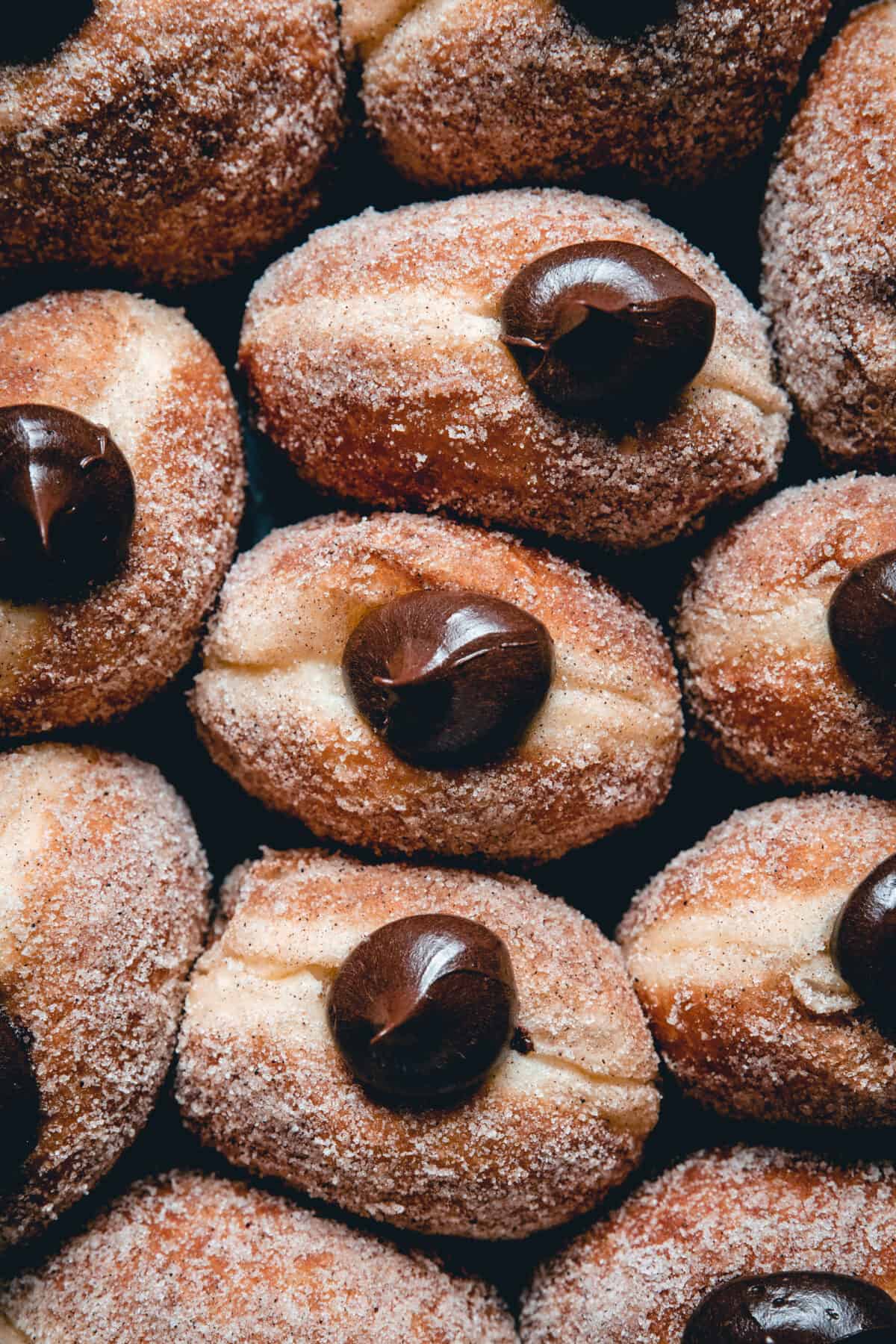This vertical, close-up photograph displays a delectable arrangement of pastries that appear to be light brown, possibly fried, and generously dusted with granular sugar. These treats, reminiscent of peanut butter cookies with chocolate kisses on top or small jelly doughnuts, encase a rich, chocolate filling that oozes out from their midsections. Approximately a dozen pastries can be seen, stacked and overlapping, in various shades from lighter beige to darker tan, giving a warm, appetizing contrast. The pastries, some with visible cracks and separations, highlight their enticing texture and fresh appearance, undoubtedly making for a mouthwatering sight.